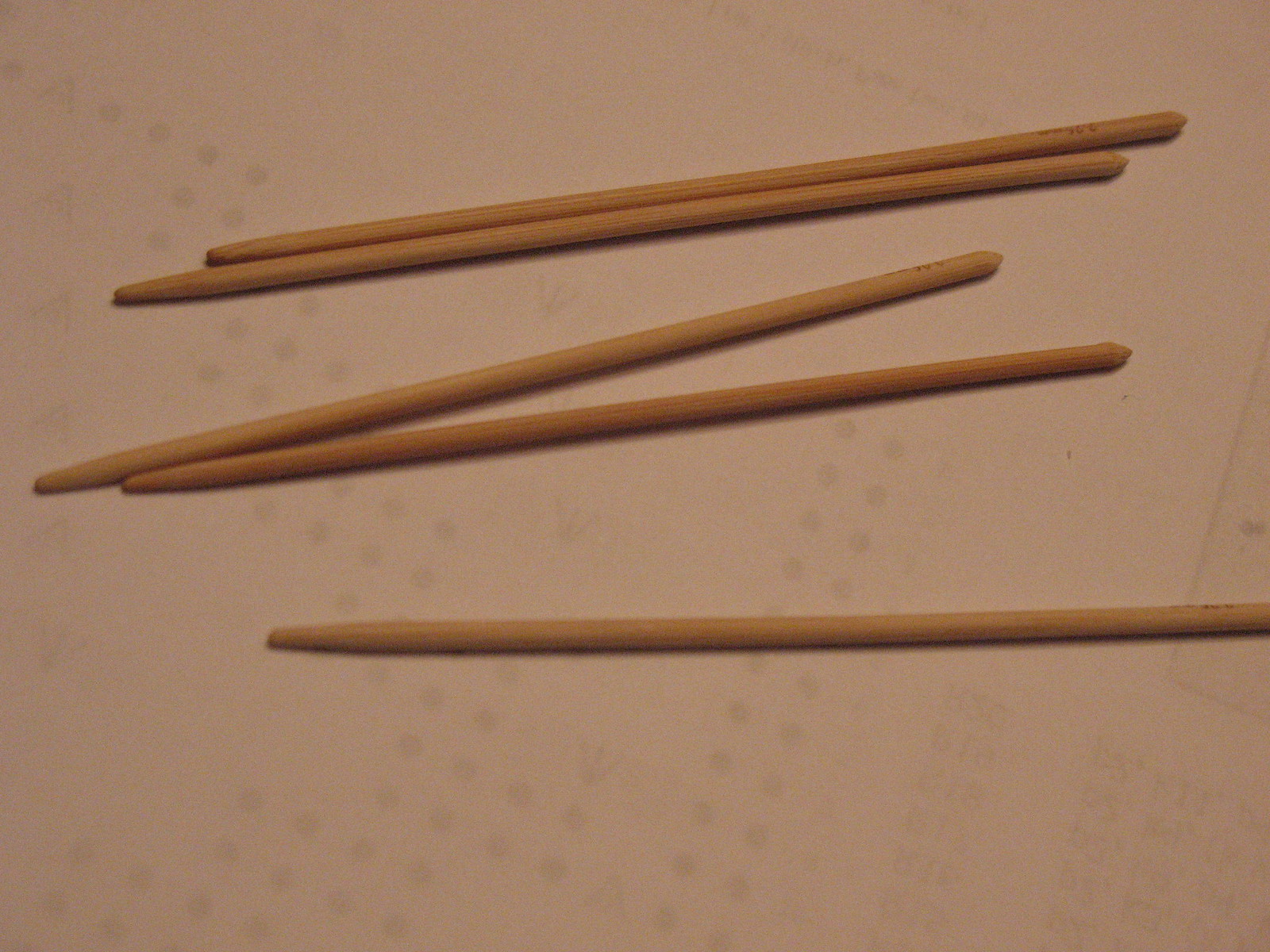The photograph depicts five slender, light brown wooden sticks, reminiscent of chopsticks, meticulously laid out on a plain white sheet of paper. The background paper faintly reveals pencil dots, lines, and indentations from handwriting on its reverse side. Each stick tapers gradually to a sharper point on the right end and a more rounded point on the left. Arranged with a subtle order, the top two sticks lie parallel and close together, the middle two are slightly touching, and the final one rests alone at the bottom. Visible on the right ends of the sticks is some type of etched writing. The detailed grain of the wood is visible, accentuating their natural texture.